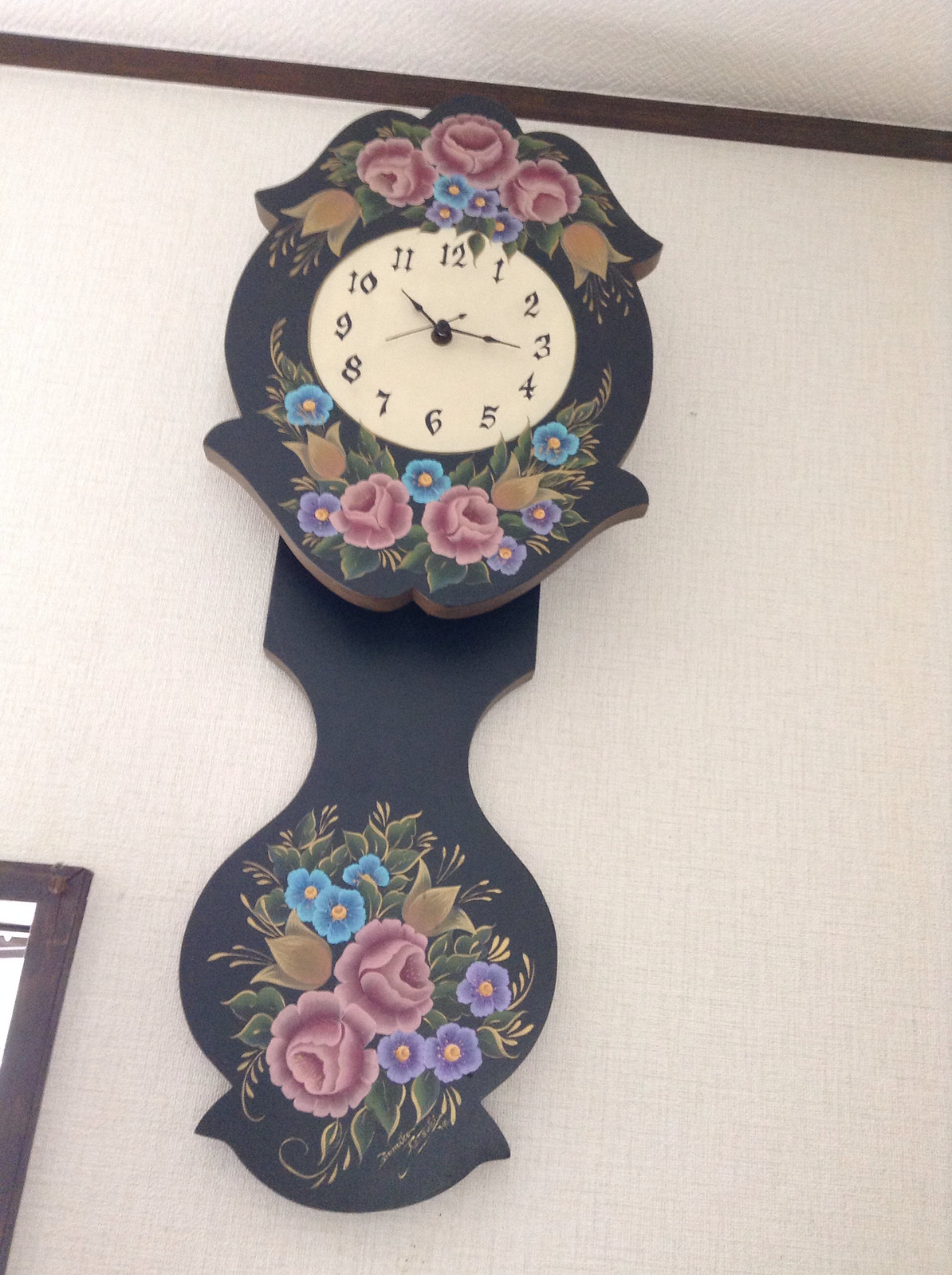This is a close-up photograph of an antique clock with a portrait orientation. The clock's face, an off-white hue, prominently features black numbers and a black dial. Surrounding the clock face is an ornately designed black frame adorned with intricately painted pink, blue, yellow, and purple flowers at the top and bottom. Below the clock, an additional ornate black piece complements the design, also embellished with the same floral pattern. This elegant timepiece is set against a white wall framed with dark brown edging, highlighting its intricate details and vintage charm.